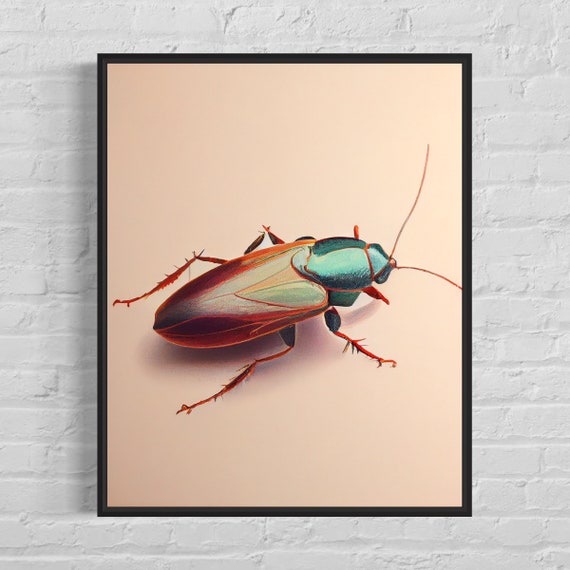A framed artwork displays a central, detailed depiction of a beetle-like cockroach against a light pink background. The image is encased in a black frame mounted on a gray wall. The insect features a multicolored exoskeleton, with a shiny, dark turquoise head and front section, transitioning into a reddish-brown and violet hue along the abdomen and wings. The legs and antennae are prominently visible, extending from both sides of its horizontally oriented body. The composition resembles a blown-up, detailed illustration of the insect, showcasing its shiny armor-like shell, spikes, and fine hairs. The background of the framed piece contrasts subtly with the pink canvas, enhancing the vivid coloration of the central figure.